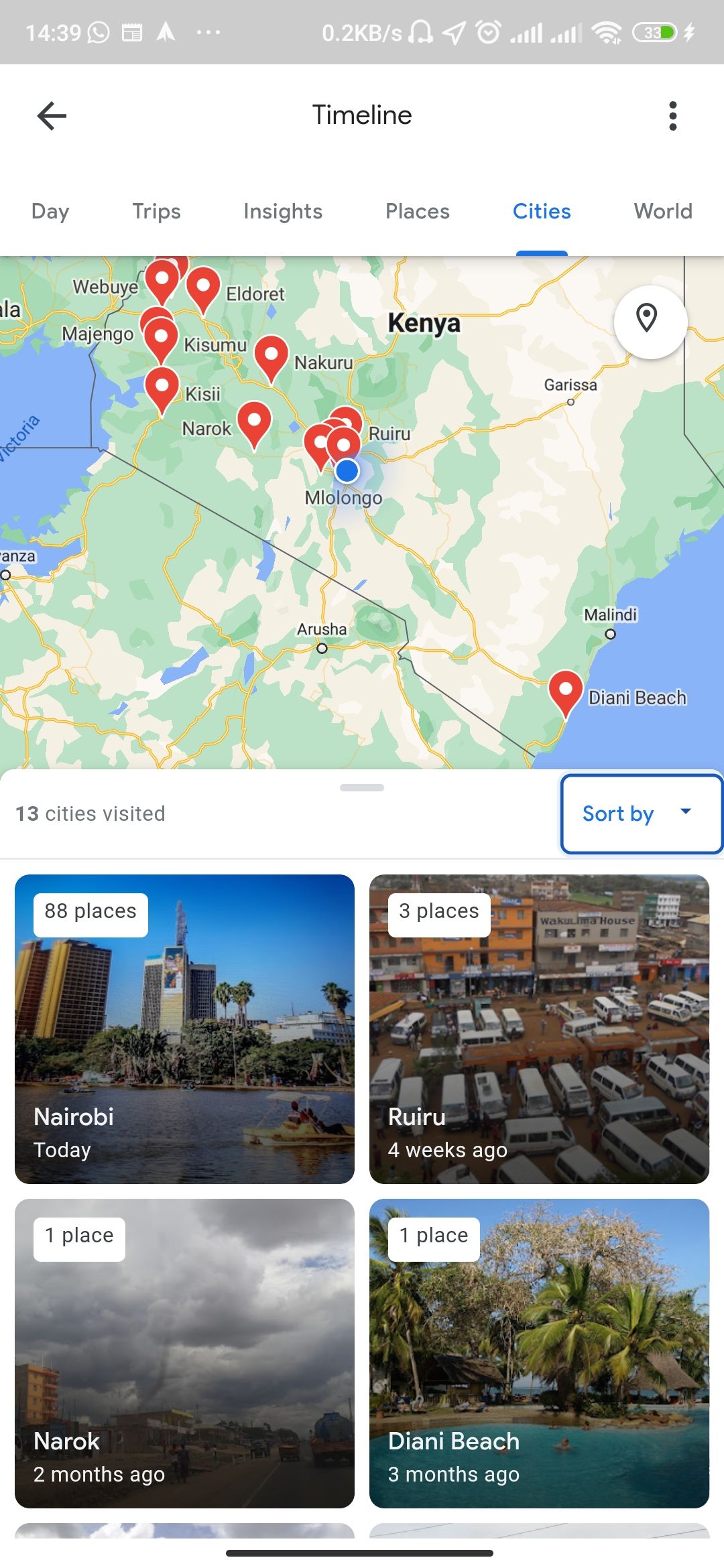This image captures a screenshot of a cell phone displaying a specific section of a travel app. The top of the screen shows various tabs labeled "Timeline," "Day," "Trips," "Insights," "Places," "Cities," and "World." The "Cities" tab is selected, highlighted by a blue line underneath and blue text.

Beneath this tab, the user is viewing a map of Kenya, dotted with red pins each featuring a white circle in the center. These pins mark various cities such as Eldoret, Kisumu, Kisii, Narok, and Diani Beach. The text indicates "13 cities visited."

Below the map, an option labeled "Sort by" is visible, followed by a list of specific visits:
- "Nairobi today" with a thumbnail image of the city and "88 places."
- "Ruai Ruai" from four weeks ago with "3 places."
- "Narok" from two months ago with "1 place."
- "Diani Beach" from three months ago with "1 place."

Though the content cuts off at the bottom of the screenshot, it implies more entries exist beyond the visible portion.